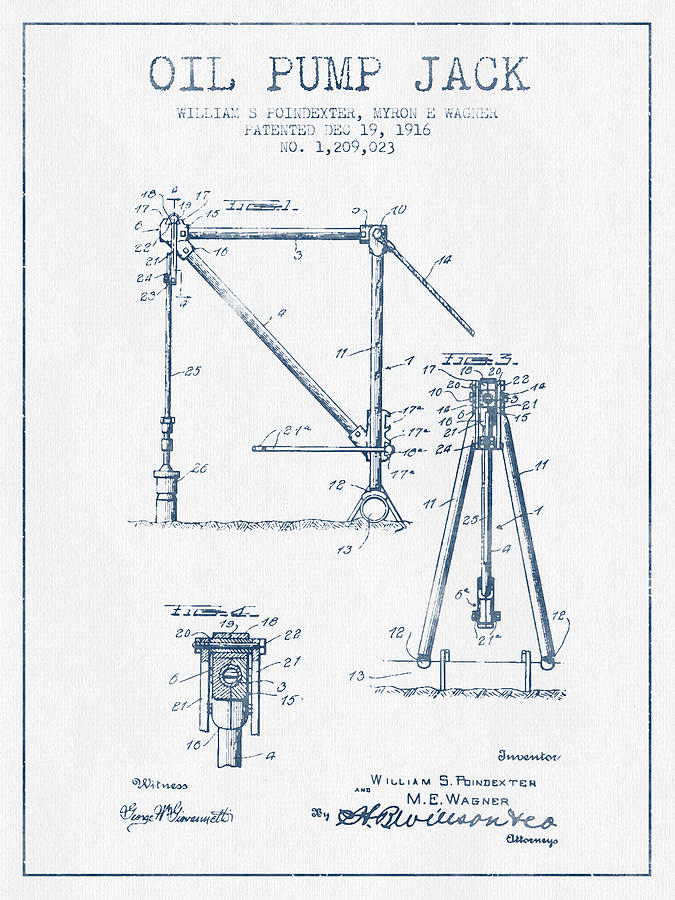This image is a vertically aligned rectangular sheet of light gray paper set against a white background, bordered by a thin black line. At the top, bold black all-caps text reads "OIL PUMP JACK." Directly beneath, in smaller text, the inventors' names, "William S. Poindexter" and "Myron E. Wagner," are listed, followed by the patent date "December 19, 1916" and patent number "1,209,023."

The central part of the paper features a detailed hand-drawn sketch of an oil pump jack, consisting of various components. On the upper left, there is a rectangular shape, while the right middle section includes a tripod-like structure. The lower left displays a smaller cylinder attached to a larger rectangular top with two bars descending on each side.

At the bottom left corner, the word "Witness" appears beneath a signature, while the names of the inventors, "William S. Poindexter" and "M.E. Wagner," and their signatures are inscribed on the lower right. The text, diagrams, and all other elements on the paper are rendered in a specific shade of blue.